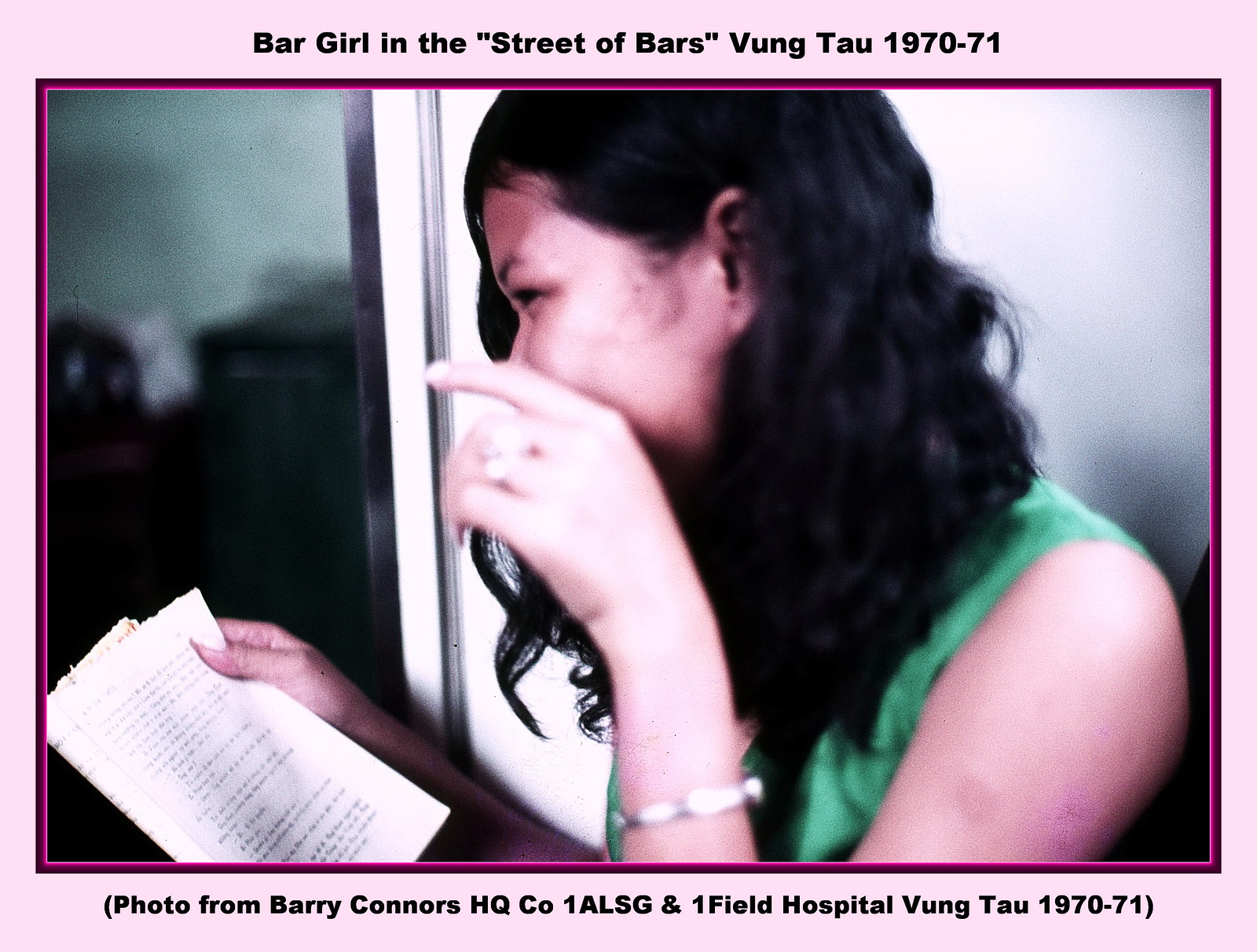In this blurry photograph framed with a pink border outlined in purplish and black hues, there is an image of a woman with black wavy hair. She is wearing a green tank top and a bracelet. The woman is partially covering her face with her hands, which are holding a piece of paper that appears to have typed text on it. She is looking sideways, perhaps with a smile, as if gazing to the left of the picture. Written at the top of the photo are the words, "Bar Girl in the Street of Bars, Vung Tau, 1970-71," while the bottom caption reads, "Photo from Barry Connors, HQ CO 1 ALSG, N1 Field Hospital, Vung Tau, 1970-71." This picture dates back to the Vietnam era in the early 1970s.